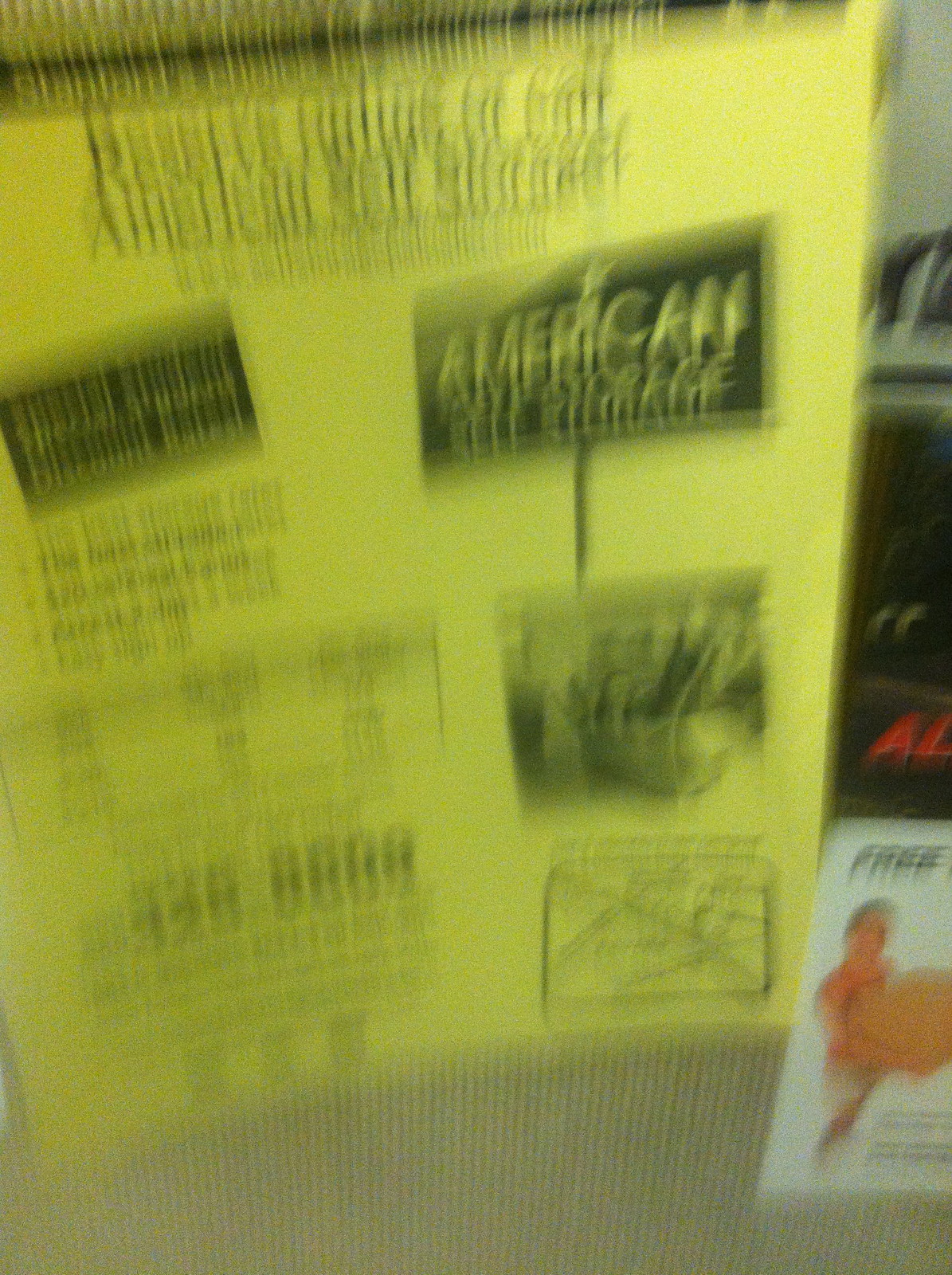The image depicts an extremely blurry advertisement on a vertically held yellow sheet of paper, which is positioned just above a tan-colored couch with a corded texture. The paper has a black border at the top and features black centered letters. At the top of the page, the title reads, "Reserve Online or Call American Self-Storage." Below this, the text "Special Student Discount Rates" is located in a rectangle on the left side, while a larger rectangle on the right displays "American VIP Storage." There are several additional elements on the paper: a small rectangular map in the bottom right, a black and white photo in the center right, and another indistinct rectangular box on the center left of the page. Partially visible in the bottom right of the photo is a business card with the words "free" and an image of a man holding a box. Despite the blurriness, a phone number can be discerned at the bottom of the advertisement. Overall, it is clear that the image showcases a promotional flyer.